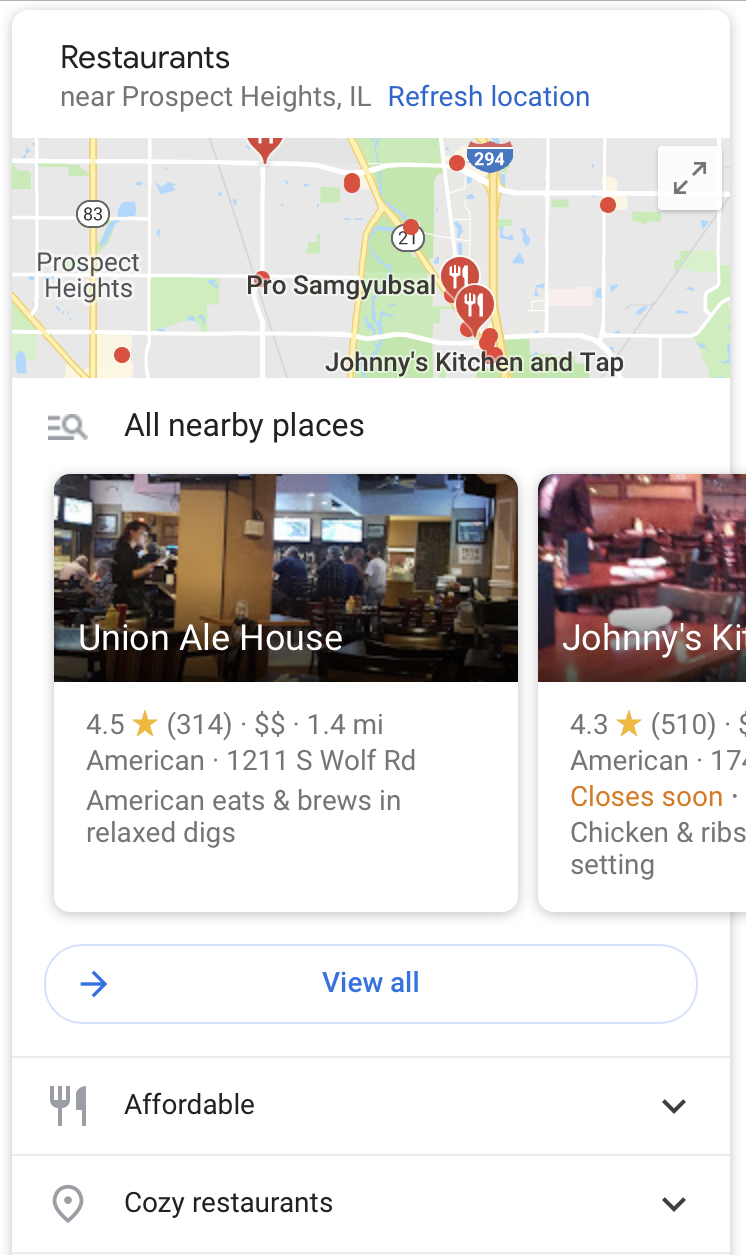A Google Maps results page for restaurants near Prospect Heights, Illinois, is displayed. On the right side, a button for refreshing the location can be seen. The zoomed-in map provides suggestions for restaurants in the area, highlighting three visible places.

Below the map, a search icon and a hamburger menu are present, accompanied by the text "All nearby places." Directly beneath this, two specific restaurant suggestions are listed. The first suggestion features Union Ale House, showcased with an image of its dining room. The listing details include a 4.5-star rating based on 314 reviews, located 1.5 miles away at 1211 S. Wolf Road. It is described as an American restaurant offering "American Eats and Brews" in a "Relaxed Digs" atmosphere.

The second suggestion is Johnny's Kitchen, also illustrated by an image of its dining room. However, the full description is cut off, revealing only a 4.3-star rating from 510 reviews, referred to as an American restaurant specializing in chicken and ribs, noted to be "closing soon."

Adjacent to these listings is a box with a right-facing blue arrow labeled "View All." Below this section, entries for affordable and cozy restaurants are indicated by drop-down arrows. The entire page provides a comprehensive overview of dining options near Prospect Heights, Illinois.